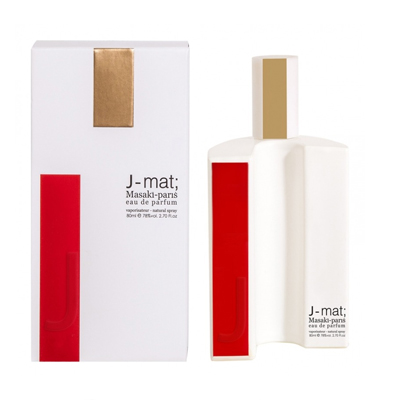The image features an advertisement for a perfume named "J.Maski Paris Eau de Parfum." On the left side of the image is a white package with distinct design elements: a red vertical stripe running up the left-hand side, a shorter gold rectangular stripe descending from near the top, and black lettering in the center that reads "J.Maski Paris Eau de Parfum." There is also some fine print below the main text that is difficult to discern. 

To the right of the package sits the actual perfume bottle. The bottle mirrors the box's design with a white body, a gold rectangle on the cap, and a red vertical stripe on its left side. The bottle's shape is unconventional, featuring a curved indentation in the center, reminiscent of a U-shape when viewed from above. This indentation gives the bottle a unique, non-standard silhouette. The same black lettering, "J.Maski Paris Eau de Parfum," is inscribed on the lower part of the bottle's white surface, accompanied by fine print detailing the volume of the perfume. This detailed styling and unique bottle shape indicate an effort to stand out in the market, suggesting a premium fragrance product.